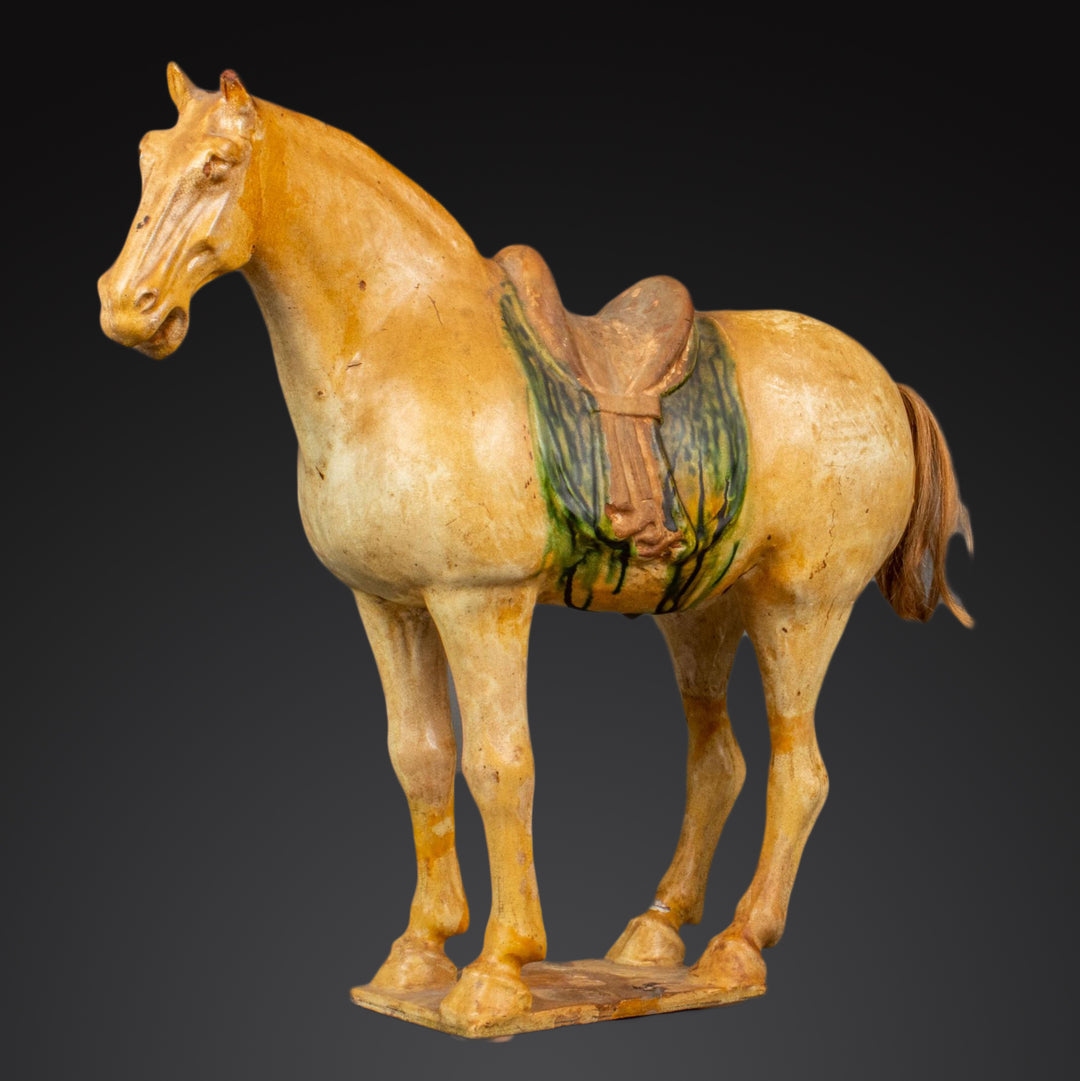The image depicts a small, intricately carved horse figurine, which appears to be made of a material that is shiny but not as glossy as ceramic. The horse is a light brown or tan color, with varying shades that include almost white highlights and darker brown shaded areas. The figurine stands on a rectangular base that securely supports all four legs. Adorning the horse is a brown saddle, complemented by a green and black blanket underneath. The horse's tail is a dark brown and seems to be crafted with realistic fiber material, giving it a natural look. Notably, the mane isn't distinctly colored but there is a visible ridge where it would be. The background of the image is a gradient of dark tones, with black at the top transitioning to gray at the bottom. The overall color palette of the photo includes shades of tan, brown, green, black, and gray, and the horse is oriented to the left side of the image.